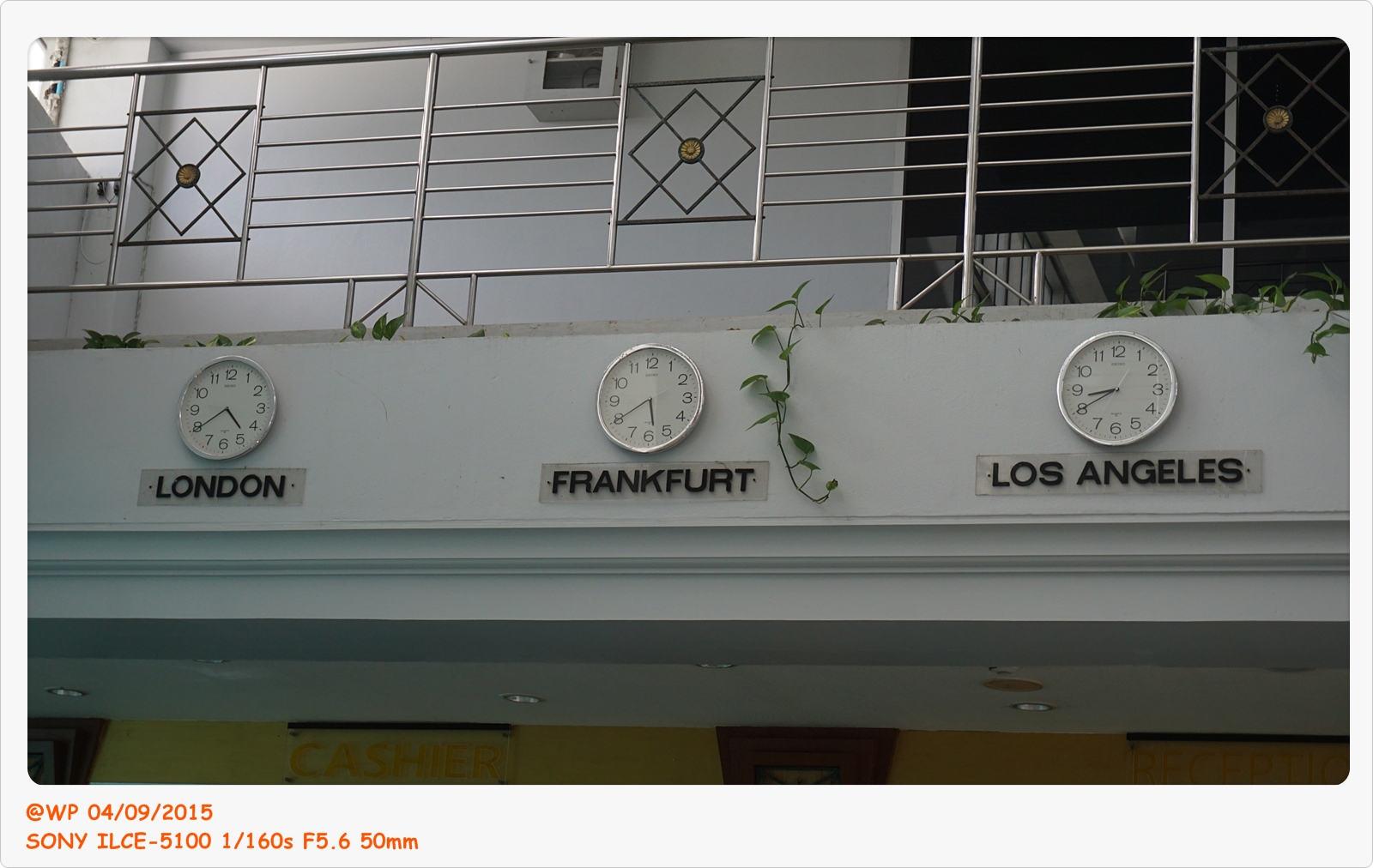The image likely depicts an airport or travel destination, characterized by the presence of three clocks on a gray wall, displaying times for different global locations. Each clock shares a uniform design: a circular shape, a silver outer frame, a white face, and black numbers from 1 to 12. The clock on the left shows the time in London, the middle one in Frankfurt, and the right one in Los Angeles.

A prominent feature at the top of the image is a metal railing, composed of silver upright posts and horizontal bars. These posts converge at square sections, each distinguished by a pattern resembling a gray-colored diamond intersected by a cross.

Surrounding the image is a white border with orange print, containing details such as a date code, "WP04-09-2015," and technical information about the camera used, "Sony ILCE-5100-1160S-F5.650mm."